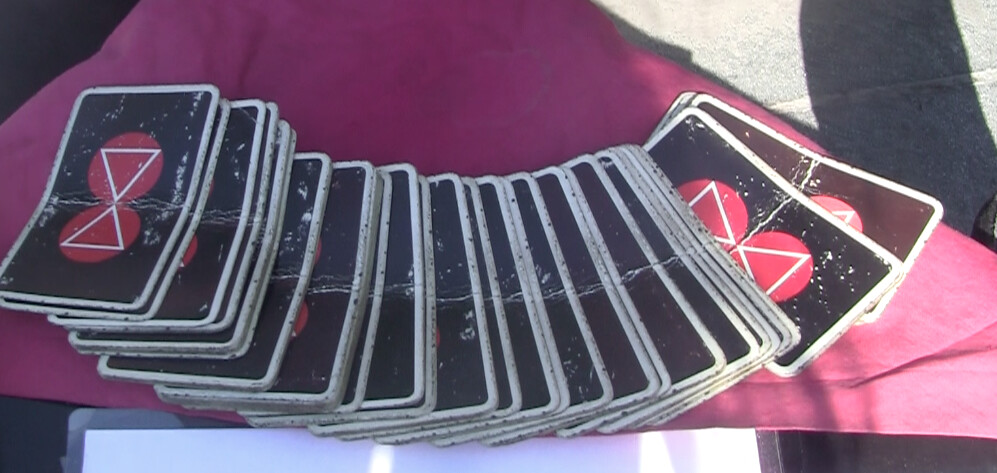In this wide, rectangular photograph, a full deck of well-worn playing cards is meticulously arranged in a curved, smiley face shape on a red tablecloth. The tablecloth, slightly folded, reveals a white piece of paper subtly peeking out from the bottom center of the image. Each card, exhibiting a distinct crease from being folded in half, features a white border encasing two central red circles. Within these circles, a white triangle outline is depicted, with the triangle tips meeting at the center where the circles touch. The cards, placed face down, obscure any symbols or numbers they might display. Adding to the scene, two concrete cinder blocks are visible in the top right corner of the photograph, contrasting sharply with the vibrant red of the cloth.